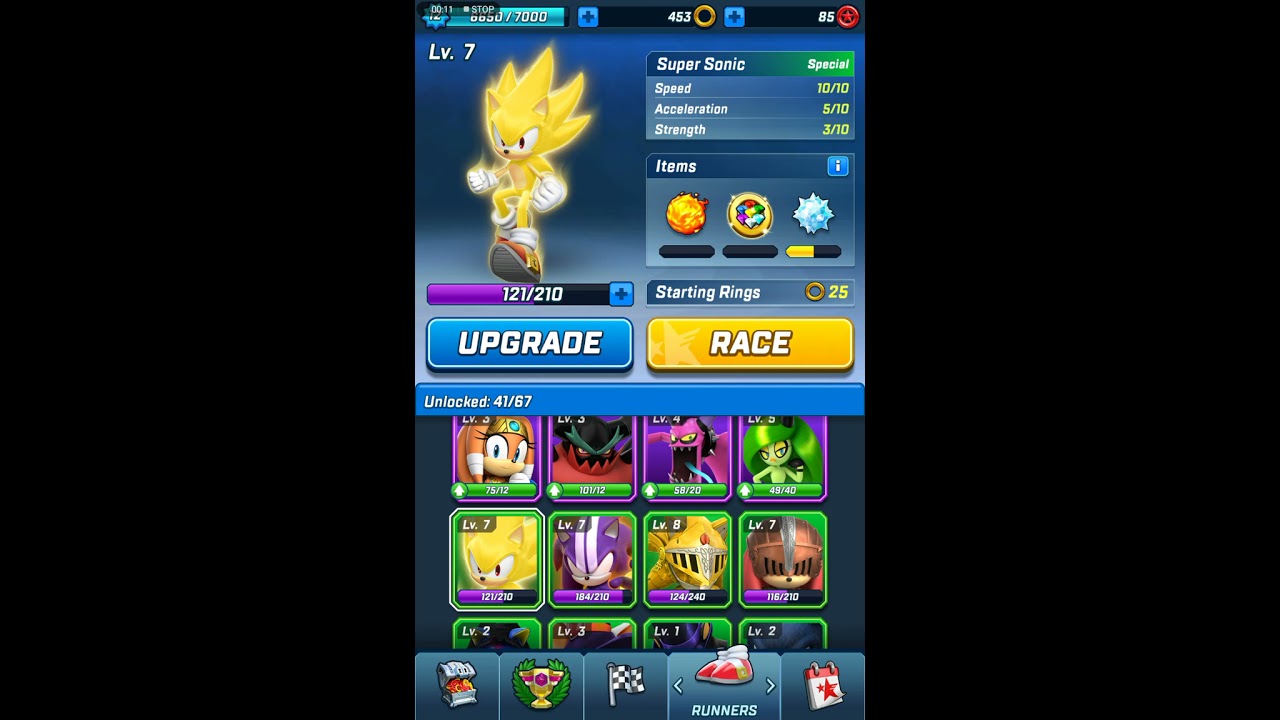The image appears to be a still frame from a high-definition video game interface, likely intended for a tablet. The central focus is a yellow character with spiky hair, black eyes, and brown shoes, reminiscent of Sonic the Hedgehog but distinctively different. On the top left, this character is depicted with a score of "121/210" beneath it, and a "blue Upgrade tab" positioned below. The right side features detailed stats: "Supersonic Special" with attributes "Speed: 10/10," "Acceleration: 5/10," and "Strength: 3/10." Below the character, there are three columns with various numerical values.

Further down, three items are depicted: on the left, a fireball, in the middle, a circular object with colorful parts in the center, and on the right, a spiked blue rock. The image is annotated with additional text, including a score of "7,000" and "453" next to a ring, and "85" next to a star, along with a "Level 7" indicator. On the bottom, there's a label for "Runners" and images of eight to twelve different characters available for selection. The entire image is surrounded by a black border, giving it a tablet-like shape, with prominent "Upgrade" and "Race" buttons in blue and yellow, respectively, situated on the left and right. The overall color palette includes black, white, pink, purple, green, gold, blue, tan, brown, red, and fuchsia.